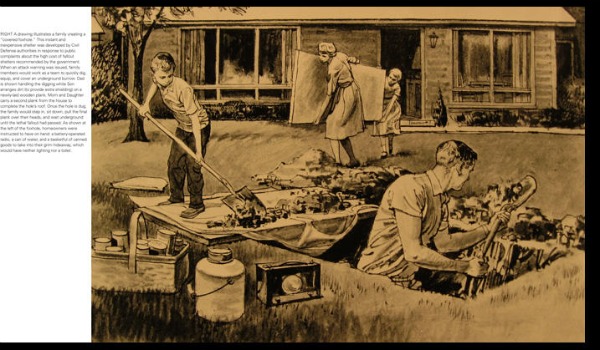The image is a page from a book, featuring a sepia-toned illustration with a yellow old paper quality. On the left one-sixth of the page is a vertical white box containing a caption in black font, which is too small to read. The illustration depicts a family engaged in the task of digging what appears to be a basement or fruit cellar in front of a house. In the foreground, the father is inside a square hole up to his torso, actively digging with a shovel. Beside him, a young boy helps by piling dirt onto a tarp spread out in front of the hole. Surrounding them are various items, including a radio, a bucket, and a basket filled with jars. In the background, a woman and a young girl, likely the mother and daughter, are seen carrying a rectangular white object out of the house. Additionally, two nurses are visible carrying a table out of the front door. A tree is positioned on the left side, suggesting a yard setting. The overall composition suggests a detailed and bustling scene of a family undertaking a practical, laborious task together.